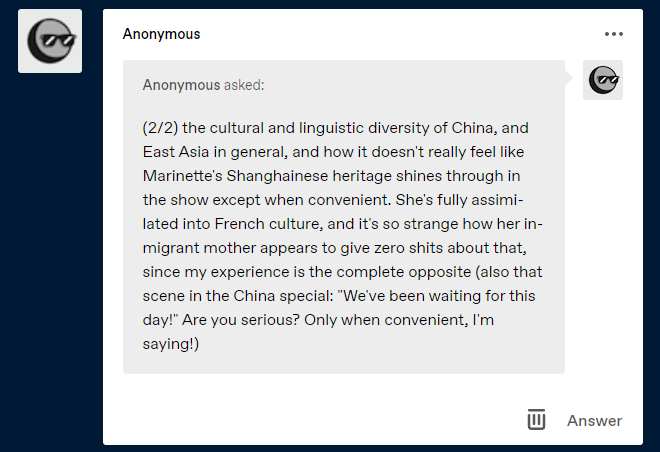The image displays a segment of a discussion board or forum where an anonymous user has posted a lengthy comment, of which we're seeing the second half. The text delves into a discussion about the cultural and linguistic diversity of China and East Asia, noting how a character named Marianne lacks evident Shanghainese heritage in a show, except when it serves a convenient narrative purpose. The user also mentions the oddity of Marianne’s in-migrant mother’s appearance. The avatar associated with the user is an illustration, not a real person, and features sunglasses and a rightward gaze. The interface is primarily dark blue, bordering on black, with options for more actions represented by three dots in the upper right-hand corner and icons for deleting the post (a trash can) and responding to it (an answer symbol) located in the bottom right corner.